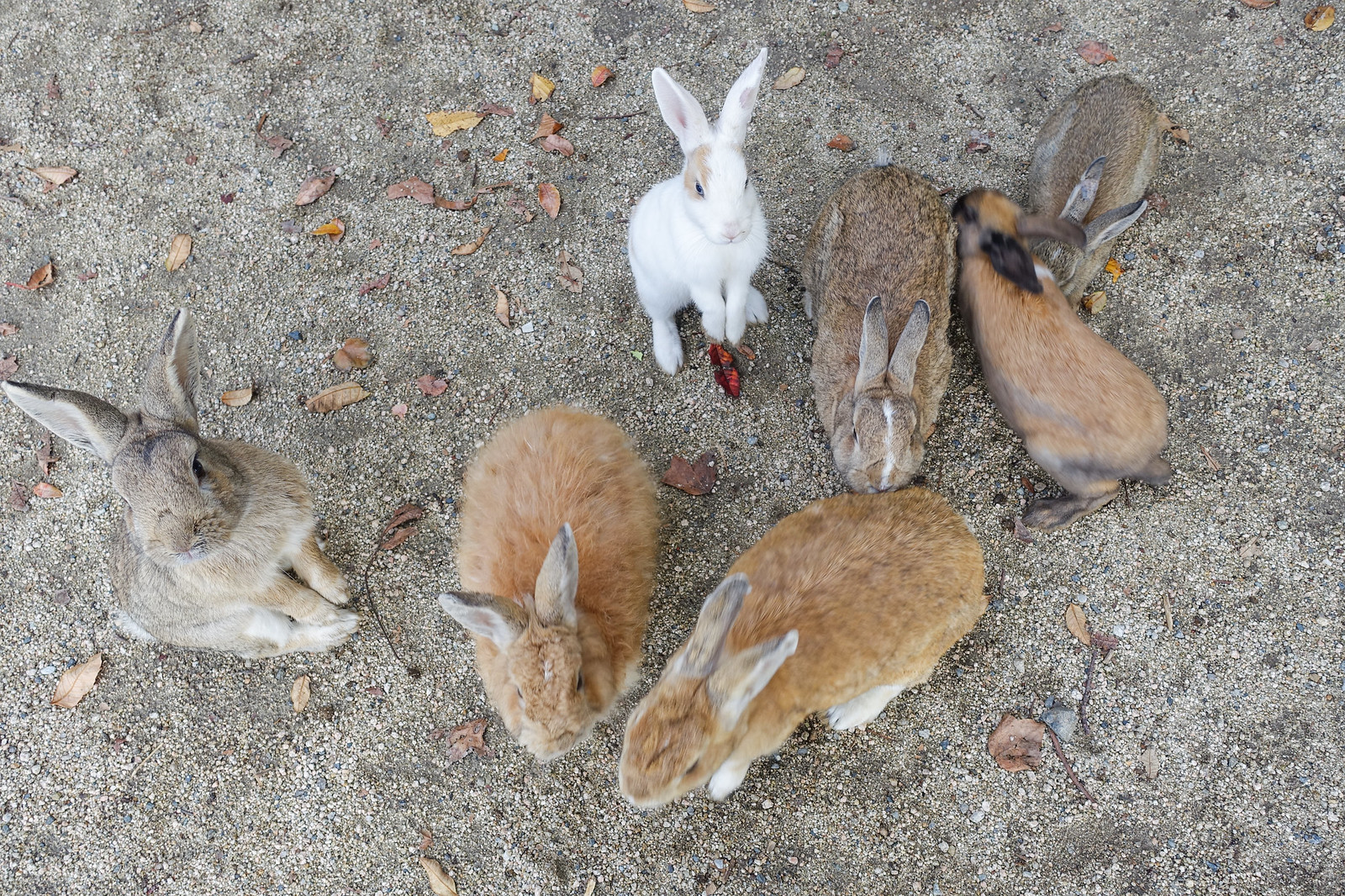This detailed color photograph captures an aerial view of seven rabbits of varying colors and sizes, positioned on a patchy, gravelly surface scattered with small, dead leaves in shades of brown and red. The scene includes a variety of rabbits: at the far left corner, a light tan or light brown rabbit stands upright on its hind legs, looking to the left with its long ears pointing straight up. Across the foreground, two light brown rabbits with white paws and shorter, gray-tinged ears face downward. Another distinct rabbit, with a predominantly white coat and brown markings around its eyes and ears, also stands on its hind legs with its paws in front and its long ears erect. Lying down to the right of the white rabbit is a brown rabbit featuring long ears folded along its back and a vertical white stripe running down its face. Adjacent to this is another rabbit, slightly blurred as if in motion, displaying a mix of brown and black fur. Nestled next to this blurred figure is a subtle, almost camouflaged rabbit with a blend of light brown and gray fur. The rabbits' positions range from upright to more horizontal, with one resting its head under another’s body. The combination of their varied postures and colors, set against the gritty terrain with scattered leaves, creates a charming and dynamic scene.